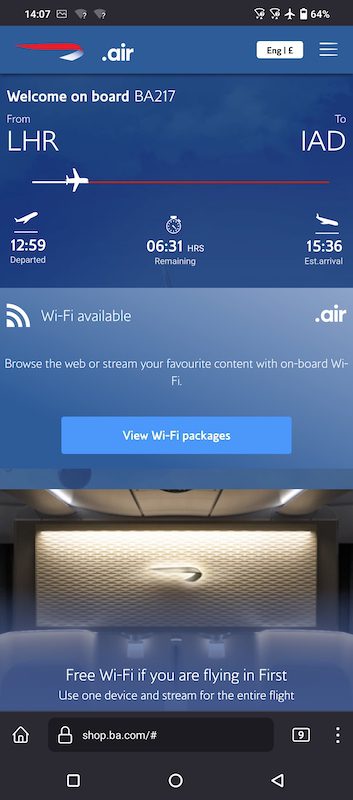This is a detailed screen capture from a smartphone, displaying information from an airline app. At the top of the screen, the current time is shown as 14:07, along with a couple of Wi-Fi icons indicating that the phone is in airplane mode, and the battery level at 64%.

The main interface of the app is visible, featuring a stylized logo of a red ribbon that curls with a white interior, labeled "ribbon.air." The upper left corner welcomes the user on board flight BA217, traveling from London Heathrow (LHR) to Washington Dulles (IAD). The flight departed at 12:59, with an estimated remaining flight time of 6 hours and 31 minutes, projecting an arrival time of 15:36. 

The app notifies that Wi-Fi is available, encouraging passengers to browse the web or stream content, and provides a link to view Wi-Fi packages. There's also an image promoting free Wi-Fi for first-class passengers, allowing them to use one device for the entire flight. Below this image, a URL is displayed: shop.ba.com for accessing the airline's online shop. The standard smartphone control icons are located at the bottom of the screen.